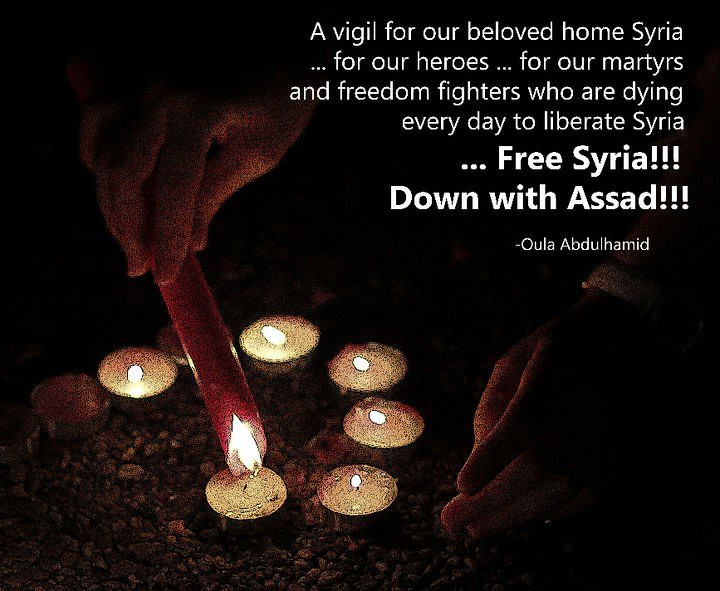In this evocative image, the surrounding darkness is punctuated at the bottom left by a semi-circle of tea candles being lit with a longer red stick candle held by a pair of hands. The tea candles, encased in silver lining, number seven in total; six are already lit, casting a gentle glow, while one remains unlit, partially hidden behind the red candle. At the top right of the image, a poignant quote in white text reads, "A vigil for our beloved home Syria... for our heroes... for our martyrs and freedom fighters who are dying every day to liberate Syria." Below this, in larger, bolder white text, it says, "FREE SYRIA!!! DOWN WITH ASSAD!!!" Finally, in smaller white text, the quote is attributed to Uala Abdulhamid.